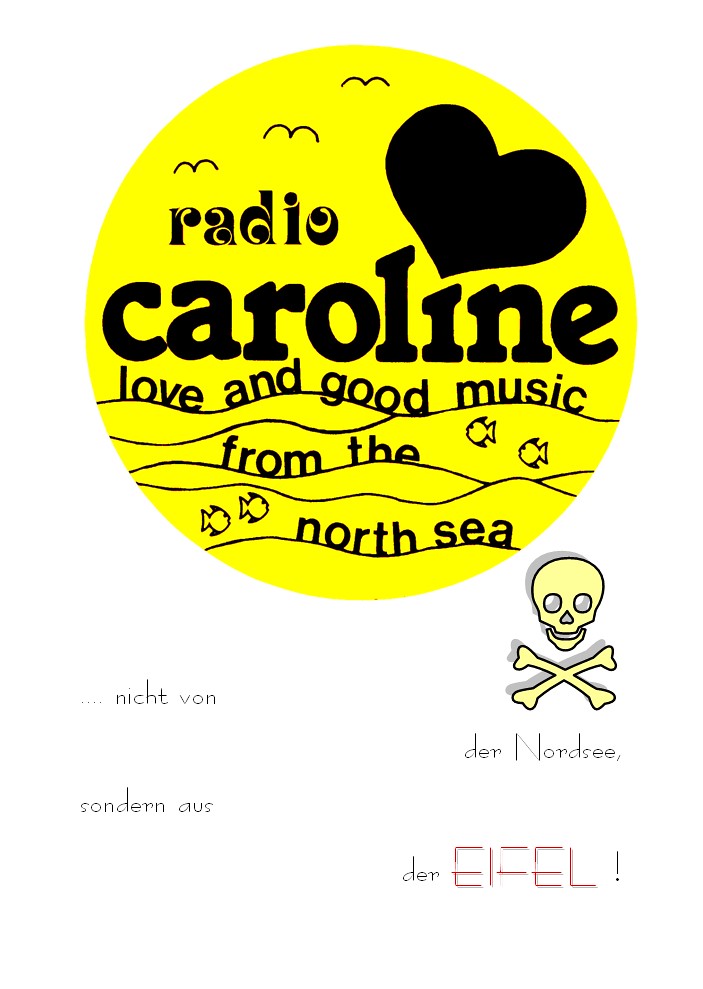The image features a white background with a prominent yellow circle at the top. Inside this circle, there is black text and illustrations. The top of the circle contains three crude drawings of birds, likely seagulls, on the left. Directly beneath these birds, the text reads "Radio Caroline" in bold black letters, with a large heart situated above the letter "i". Below "Radio Caroline" is a line of text that says "love and good music from the North Sea." The next line reads "in flow of the ocean." Beneath this line, there are illustrations of two fish, and then the phrase "two fish" appears again along with another pair of fish images. The last line within the yellow circle contains text in German, "Der Nord See."

Outside the yellow circle, there are additional details: a skull and crossbones is depicted in a pale yellow hue. Surrounding this, several phrases appear in different orientations and colors. To the left are the words "Nikt Von" and "Saudernaus" in black. On the bottom right, the text "Der" is written in black, while in red and black, the letters "FL" are inscribed. The entire image is peppered with elements related to sea life and themes of radio broadcasting, combined to create a nautical, musical motif.